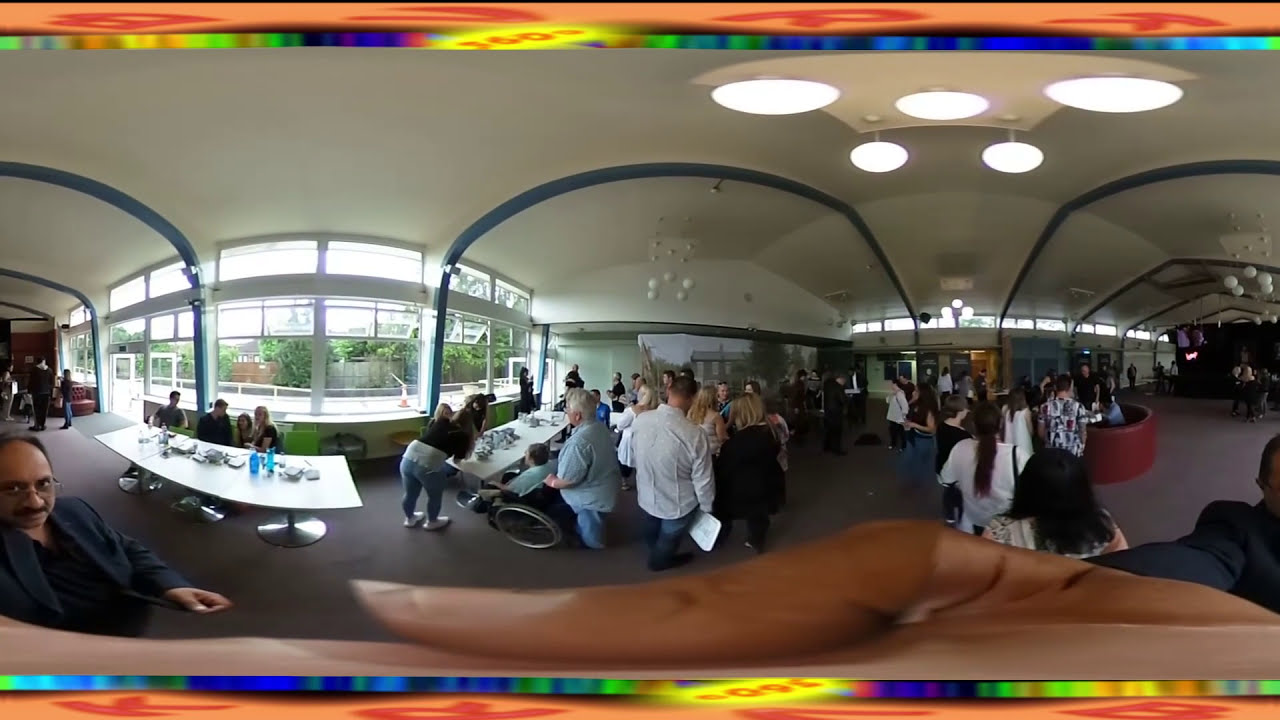The fisheye lens photograph captures a busy scene at what appears to be a convention center or large gathering space, teeming with people of all ages. The image has a rainbow-colored border with an orange stripe and the number 160 appearing in places, but is distorted by a large, intrusive finger from the photographer. The room is spacious with a white, arching ceiling dotted with round lights, and large windows along one wall.

In the left corner, a man with dark features in a black suit, black shirt, and round glasses faces the camera. In the center, an elderly lady in a wheelchair is visible, surrounded by a diverse crowd ranging from children to seniors, many wearing variously colored shirts. The right side shows more people, some seemingly in a queue, adding to the hustle and bustle of the setting.

Overall, the image is chaotic and lacks a clear theme or focal point, with the photographer's distorted hand visible at the bottom, inadvertently capturing his own arm and face.